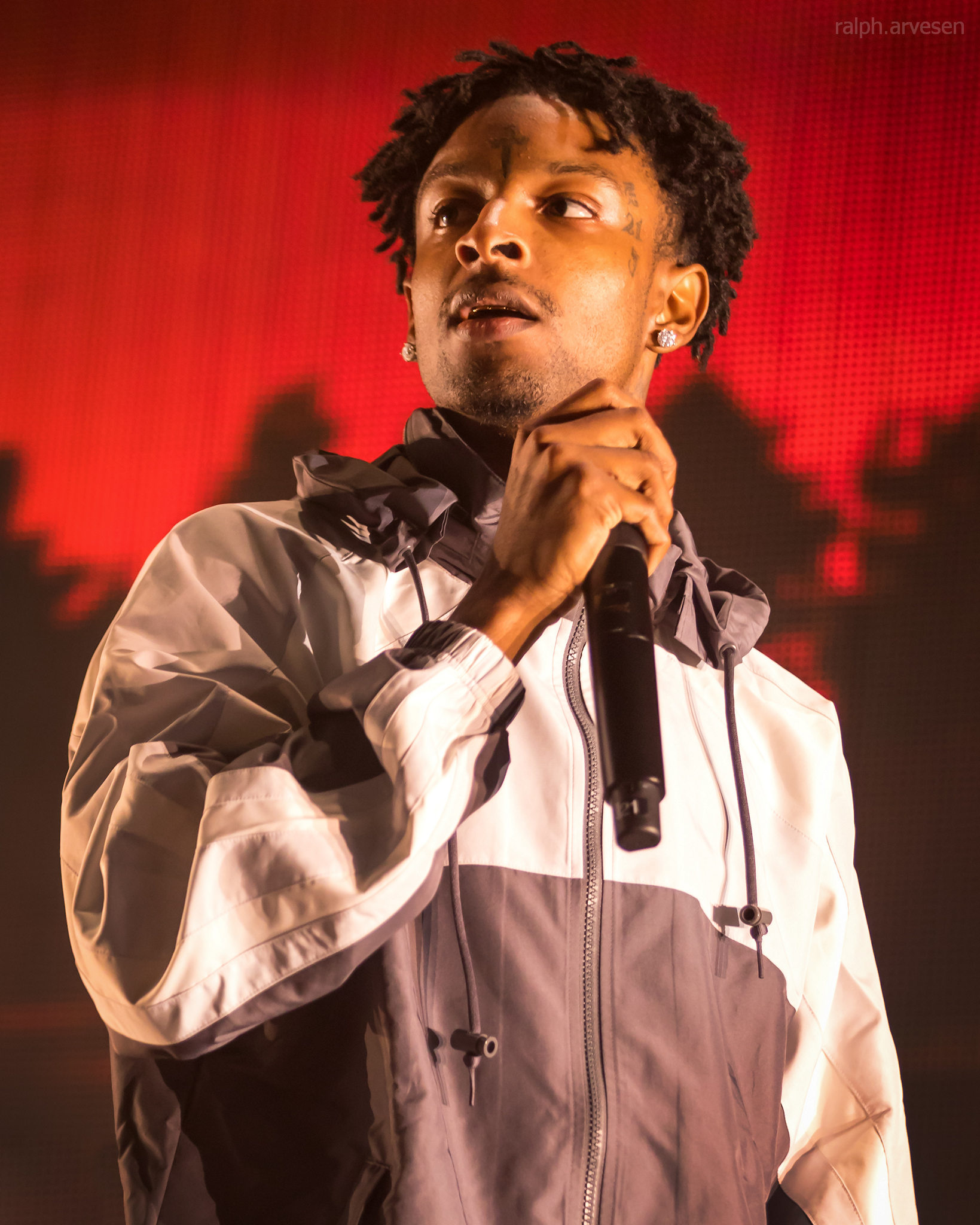In this photograph, we see the rapper 21 Savage captured mid-performance. He is holding a black microphone in his right hand and is looking off toward the upper left, seemingly focused on something in the distance. He is dressed in a light gray and white windbreaker, zipped up, which complements his stage presence. His face is adorned with notable tattoos, including a cross between his eyes above his nose and the number "21" next to his left eye. He has two large, round stud earrings in each ear, and his facial hair consists of a neatly groomed stubble covering his chin and upper lip, along with a hint of a mustache.

The background is a blur of red and black, appearing somewhat pixelated or textured, adding a dynamic and somewhat mysterious element to the overall scene. This ambient backdrop is likely a screen with moving graphics that enhance the live performance atmosphere. At the very top right of the image, the name "Ralph Arvesen" is translucently overlaid, crediting the photographer. 21 Savage's short dreadlocks, facial tattoos, and signature style make him instantly recognizable, and this snapshot effectively captures the intensity and energy of his stage presence.